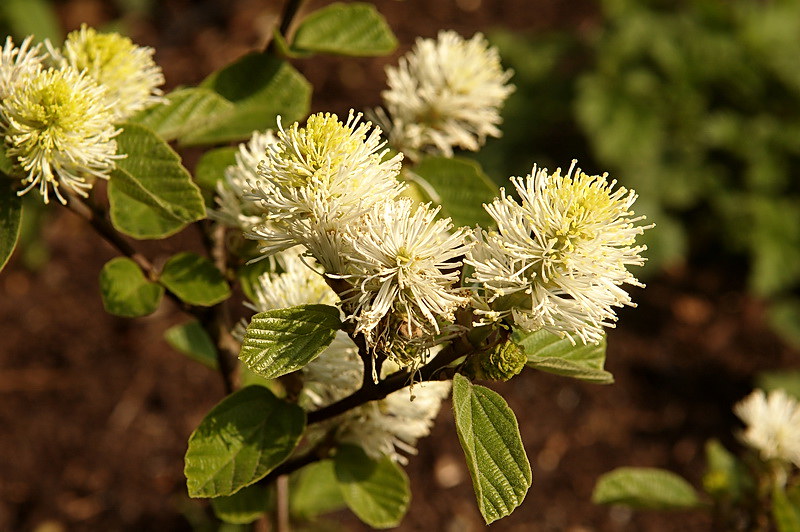This image features a close-up of a cluster of ten white flowers with yellow centers, prominently positioned in the center of the frame. Despite their spiky appearance, the flowers seem to be wilting and drying out, with parts turning brown and becoming extremely thin, indicating neglect and difficulty surviving. Some of the lower sections of the flowers are visibly dying, contrasted by the very green and alive leaves surrounding them. The background is unfocused and features brown sticks and other unclear elements on the ground, enhancing the overall theme of decay against a backdrop of vitality.